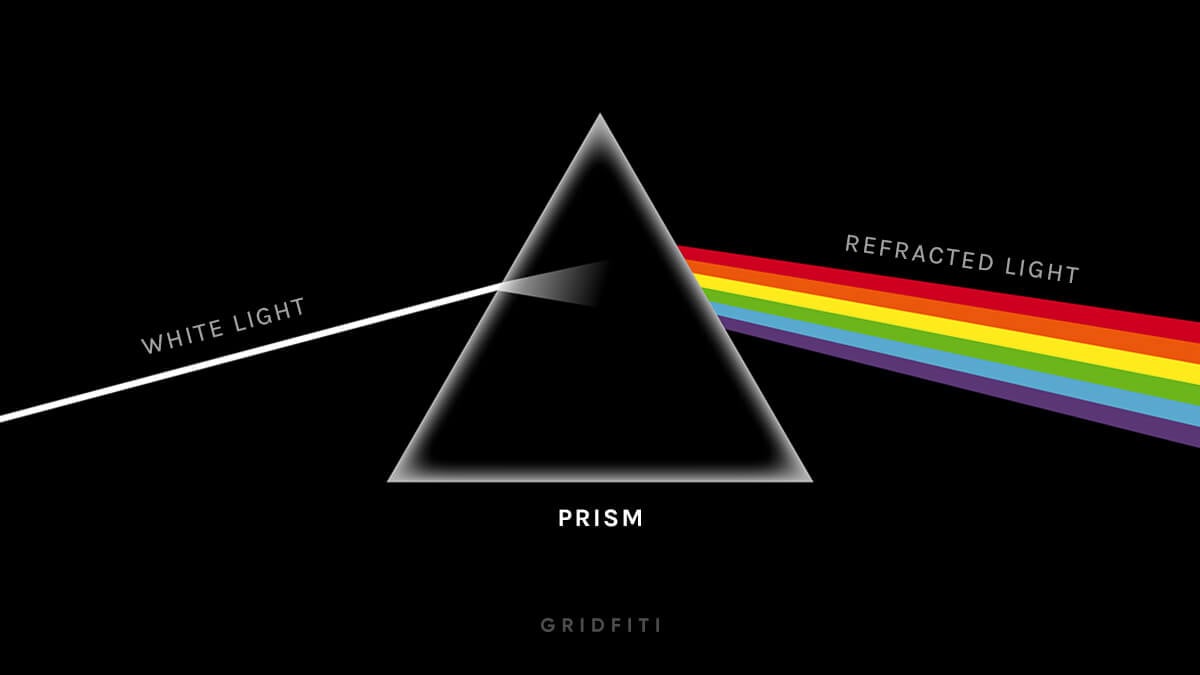The image is a detailed visualization of how white light is refracted. Set against a black background, the graphic prominently features a triangle-shaped prism with a gray outline located centrally. On the left side of the prism, there is a white beam of light labeled "white light," which enters the prism. As the light passes through, it refracts, splitting into various colors. Emerging from the right side of the prism, this refracted light fans out into distinct lines of red, orange, yellow, green, blue, and purple, collectively labeled "refracted light." Beneath the triangle, the word "PRISM" is clearly written in white capital letters. At the bottom of the image, the designer's name, Gridfiti, is subtly displayed in light gray text, adding a professional touch to the illustration.